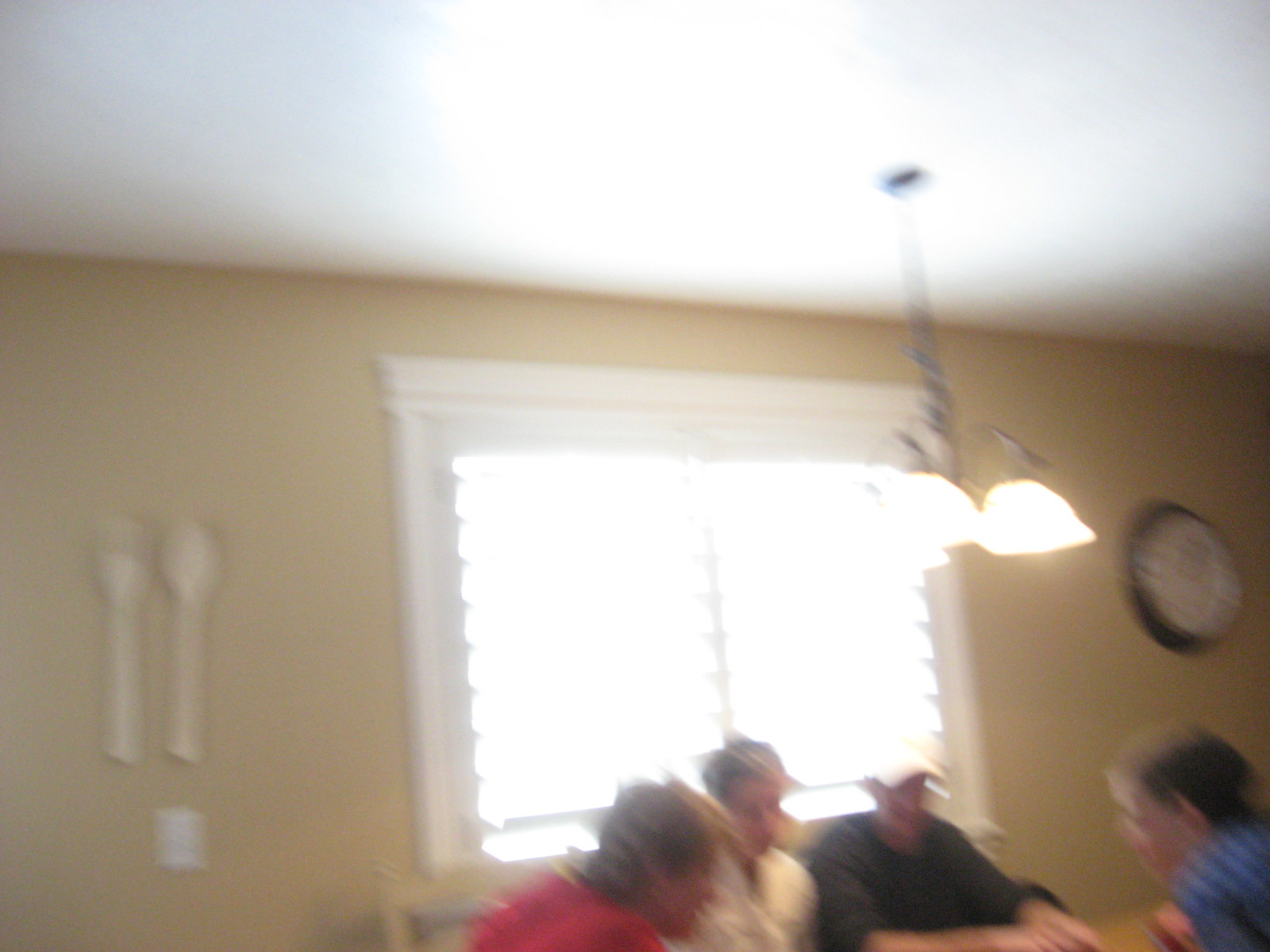A group of people is gathered around a table in what appears to be a kitchen or dining room. On the left side, there is a man wearing a baseball cap, dressed in a brown shirt. Next to him, a woman in a white top is seated. At the far end of the table sits another individual in a red top, with short brown hair, whose gender is not easily identifiable. Across from them, there is either a child with short brown hair or a man wearing a blue top. The setting is bright, thanks to a chandelier above the table, adorned with large glass globes, providing ample light.

Behind them is a window covered with large wooden blinds. The room has a tan-colored wall, decorated with oversized spoon and fork ornaments. A large clock with a white face and black trim is mounted to the right side of the window, completing the cozy and well-decorated ambiance of the room.